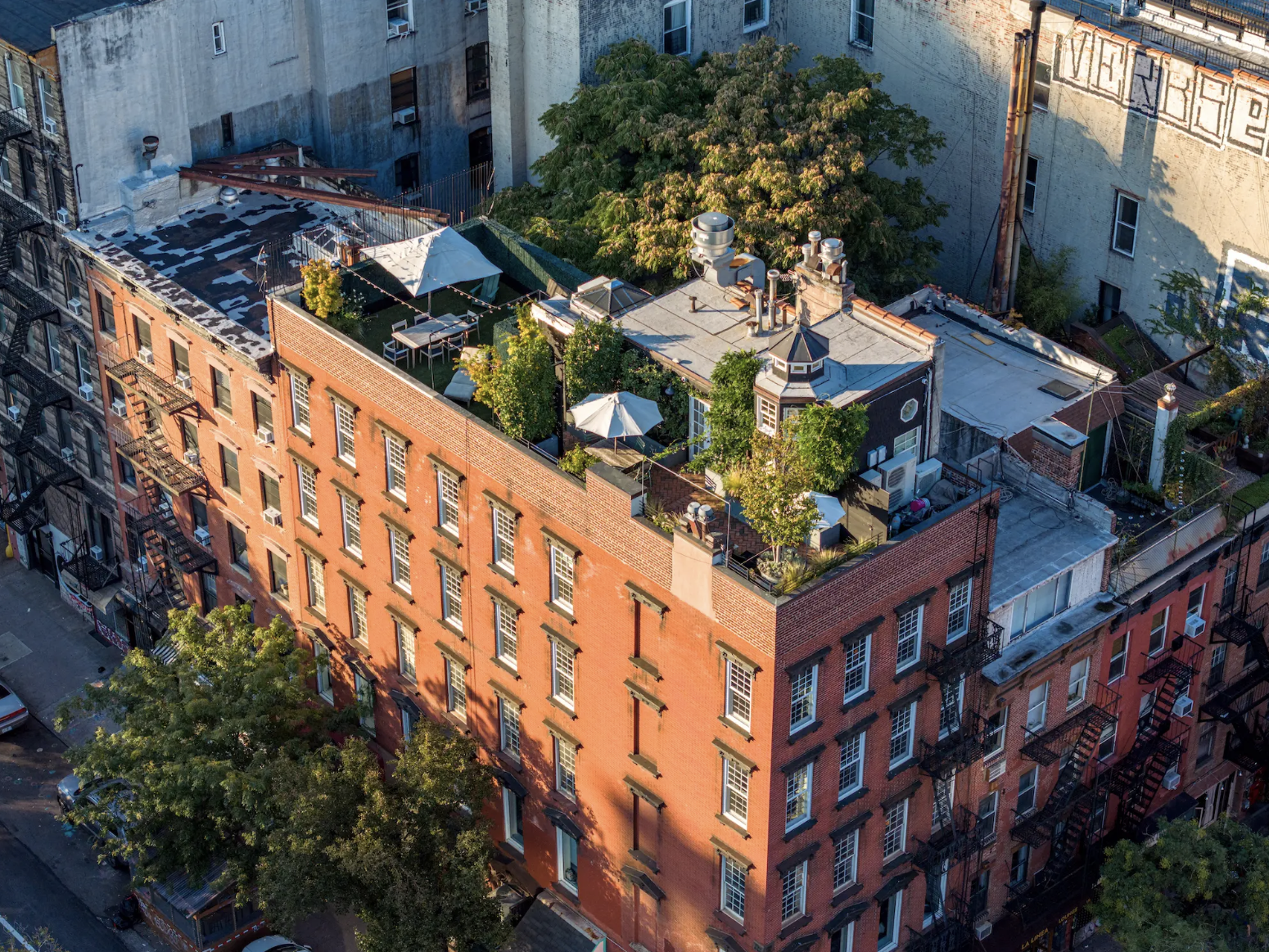The image depicts an elevated or aerial view of a large corner red-brick apartment building, likely located in a city. The building has four to five floors and features fire escapes on both the left and right sides. The structure has graffiti at the top and air conditioning units attached. The rooftop is notably detailed with a lush green garden area, including various potted trees, bushes, and an umbrella positioned over a table, suggesting an outdoor seating area. Additionally, there is a small turret or mini spiral tower and a white door that leads into this rooftop garden. The building is adjacent to a shorter structure with a plain roof and is surrounded by more buildings with varying colors, including white and gray-yellow walls. The image also captures trees both growing inside and around the buildings, along with a sunlit gray sidewalk below with scattered green trees.